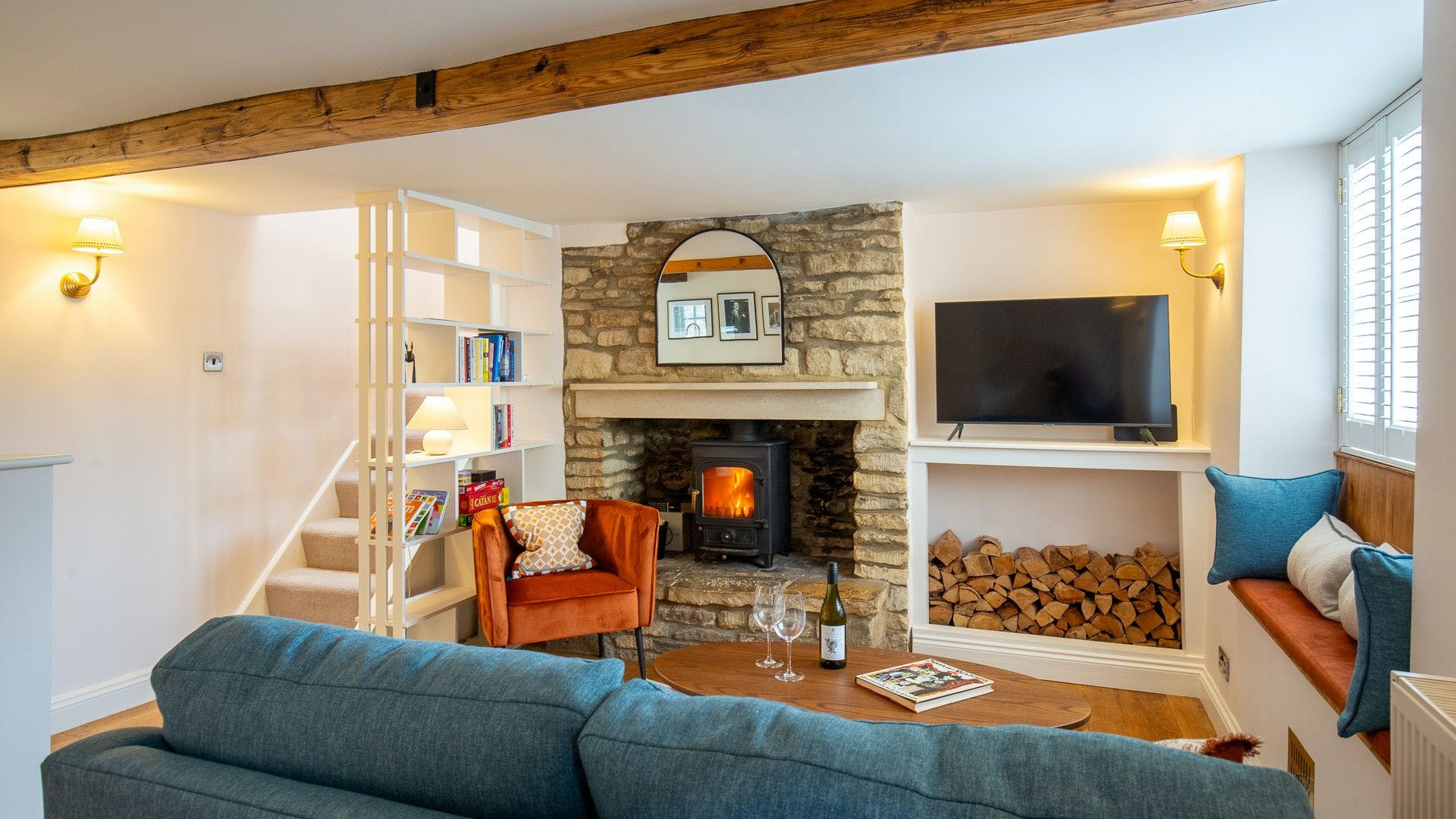The image showcases a vivid, inviting living room that blends rustic and modern decor. On the left side, a staircase descends into the room, flanked by a transparent bookshelf. An orange chair sits cozily near the base of the stairs. Dominating the center is a robust rock wall encasing a dark metal fireplace, where logs burn warmly. Above the fireplace and to the right, a flat-screen TV is mounted, with a neat white cubby beneath housing more logs. Adjacent to this setup, a window with a cushioned bench lets in daylight, adding brightness to the space. The room's warmth is complemented by a deep blue couch adorned with matching throw pillows, facing a polished wooden oval coffee table at the center. This table holds a book, a bottle of wine, and two wine glasses. Overhead, a decorative wooden beam crosses the ceiling, adding a charming finishing touch to the room's aesthetic.